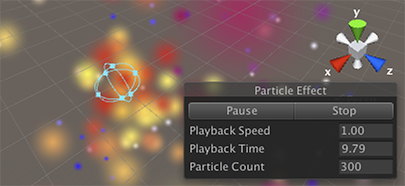The image appears to be a low-resolution screenshot, likely from a video game or an app, featuring various controls and visual elements on a grid plane background. The primary colors visible are dark gray for the background and light gray for the grid. Scattered across the grid are glowing circles or dots in red, yellow, purple, blue, and pink. On the left side, there is a bluish object resembling a circular wireframe. In the upper right corner, there is a geometric compass showing the X, Y, and Z axes, rendered in green, white, blue, and red. 

In the lower right corner of the image, there is a settings or utility box titled "Particle Effect." This box is divided into two columns: "Pause" and "Stop." Under "Pause," there are three adjustable parameters: playback speed (1.00), playback time (9.79), and particle count (300). The rest of the image is somewhat blurred, with noticeable splashes of purple, yellow, and orange colors in the background.